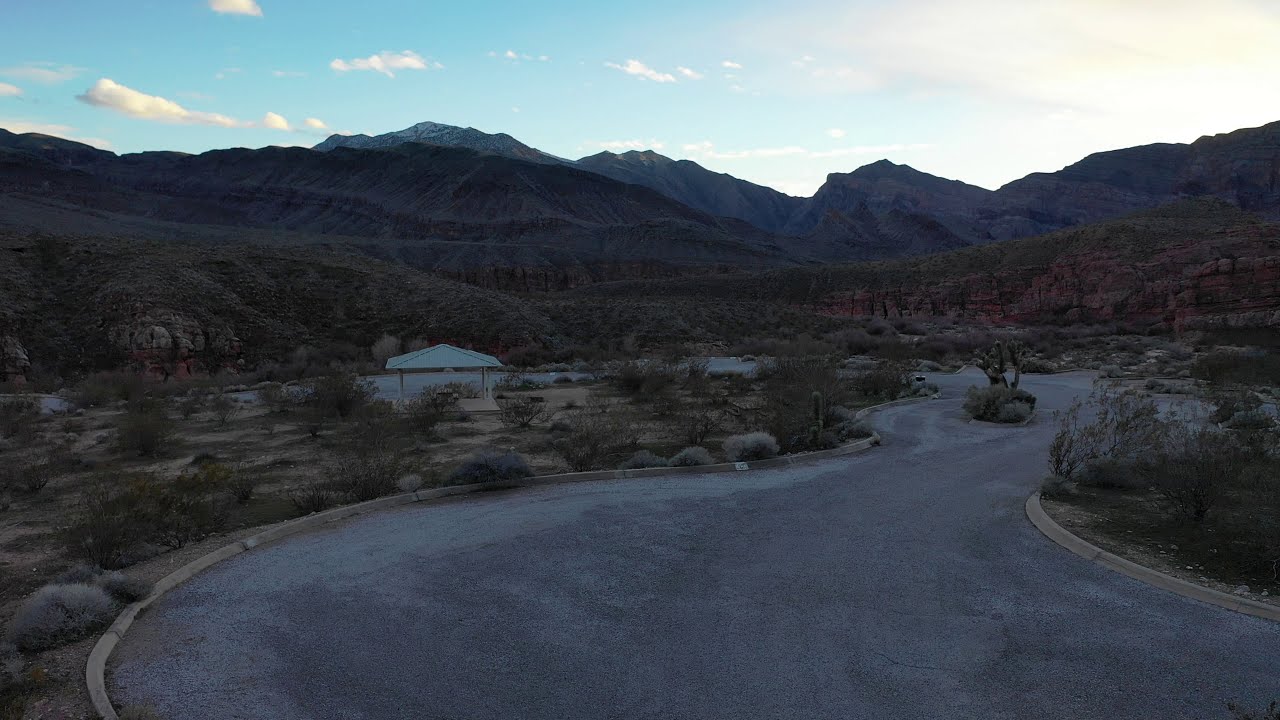The image depicts a serene desert landscape under a mostly clear, blue sky dotted with thin, fluffy white clouds. In the background, tall, rocky mountain ranges colored in grey, brownish-tan, and reddish hues stretch across the horizon, adding rugged beauty to the scene. The camera angle suggests a ground-level perspective, capturing the vast expanse of sandy ground and sparse desert foliage, including cacti, bushes, and dry-looking trees with various shades of green and brown stems.

Dominating the foreground is a winding asphalt road, empty and gradually narrowing as it stretches toward the horizon. The road curves gently and is flanked by patches of grass and dirt, with a clear boundary of pavement separating them. At one point along the road, a white canopy or pergola is visible, possibly serving as a rest stop, and is supported by four poles. Adjacent to the pergola is an empty parking lot, devoid of any cars.

The lighting in the image suggests it might be evening, with the sun potentially setting and casting a warm glow over the landscape. To the right, the sky is very bright with more pronounced white clouds, while the left side remains clearer, showcasing small clouds. The scene exudes tranquility, with the natural desert elements emphasizing the solitude and expansive beauty of the environment. There is no text within the image, allowing the viewer to fully immerse in this captivating desert setting.